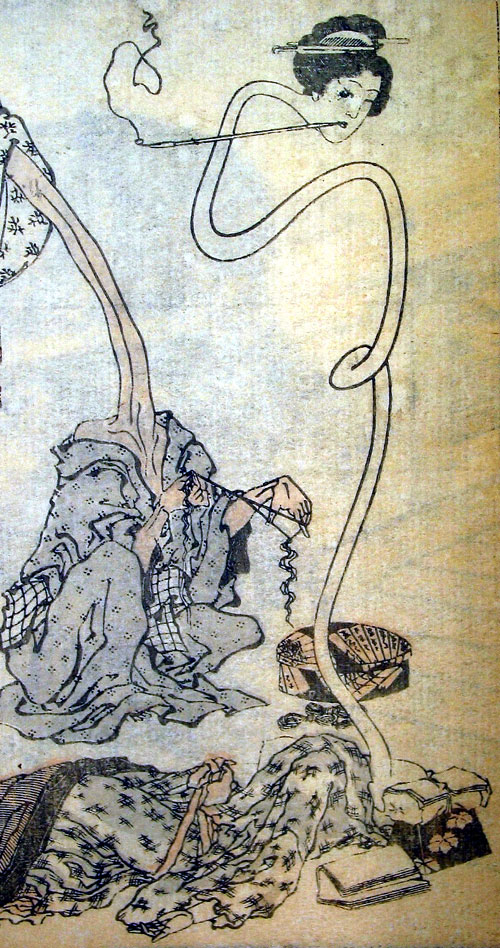The image is an intricate Japanese-style illustration featuring surreal, elongated necks and traditional elements, rendered in pen and ink with subtle color shading such as dull blues, tans, and whites. Central to the scene is a traditionally dressed Japanese woman with her hair elegantly tied up, smoking a long pipe, and playfully winking. Her neck stretches absurdly long, akin to a comic book or a snake-like spiral, creating a fantastical and almost eerie appearance. Below her head, her kimono lies strewn on the ground, suggesting a surreal extension that blends into her environment.

To the left of the main figure, another character is depicted with an unnaturally long neck, although their face is not visible. This figure is clothed in wrinkled, layered garments and appears to be performing some mysterious activity with a rope and a box, adding a mystical and unsettling dimension to the scene. The box seems to house a pattern, perhaps suggesting a connection to the snake motif. The overall composition merges traditional Japanese aesthetics with imaginative, cartoony distortion, creating a striking, dream-like visual tableau.